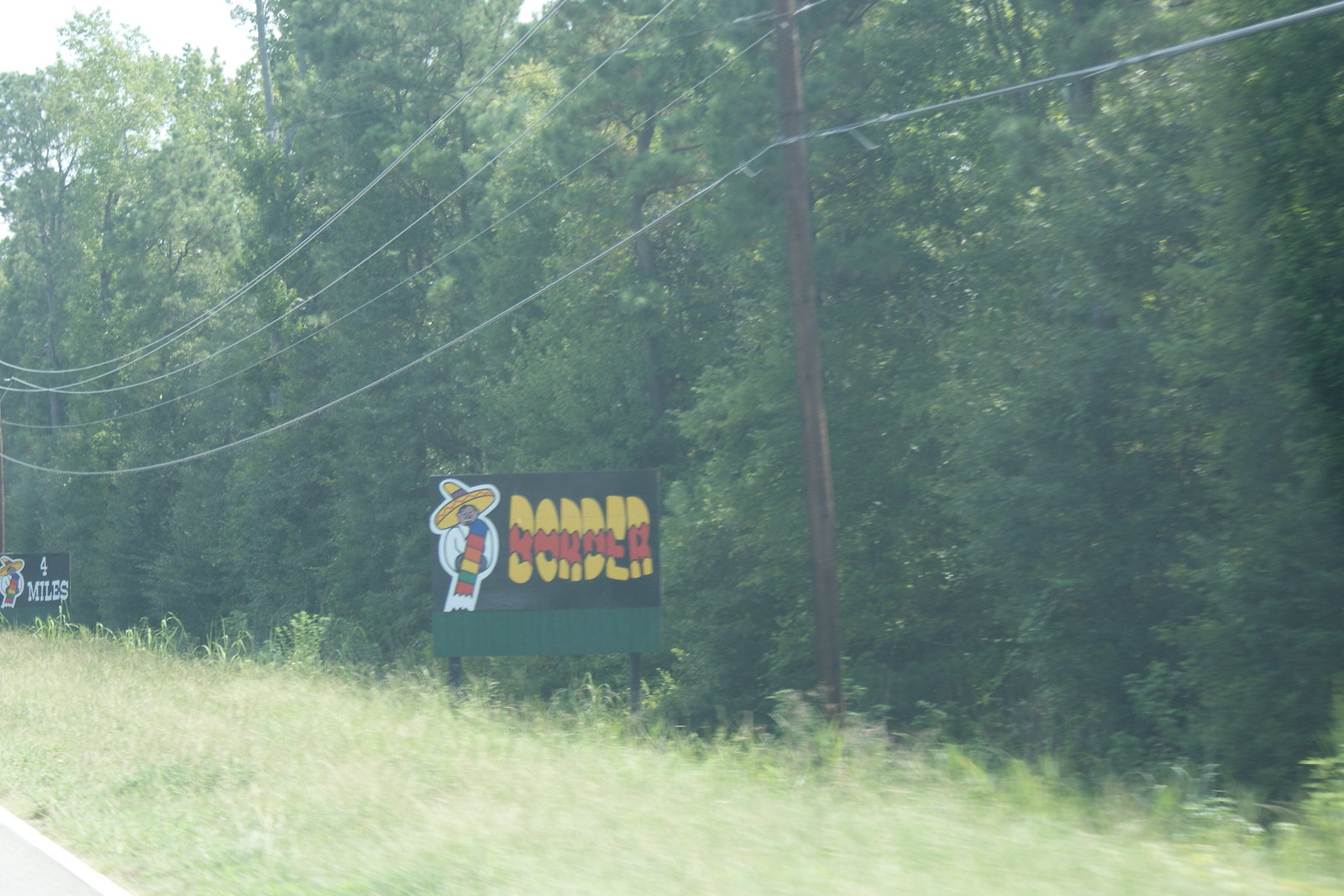The image depicts a roadside scene dominated by a small billboard-like promotional sign at its center. The prominent figure on the left of the sign is dressed in a white suit, accessorized with a large-brimmed yellow hat featuring a gray band, and a vibrant scarf draped over one shoulder in a spectrum of red, blue, orange, yellow, and green. To the right of this figure, bold red and yellow lettering spells out the word "border," with the top and bottom in yellow and the center in red, all set against a black background. Below this, a green border frames two dark legs at either end of the sign.

In the background, another sign alongside the road also features a black background and white text reading "four miles," accompanied by what appears to be the same figure in white attire on the left side. The roadside itself is unkempt, with long grass and weeds growing wild. Utility poles with sagging wires line the road, and a woodsy area with tall, lush green trees lies beyond them. The edge of the road is discernible with a white line and faded gray asphalt.